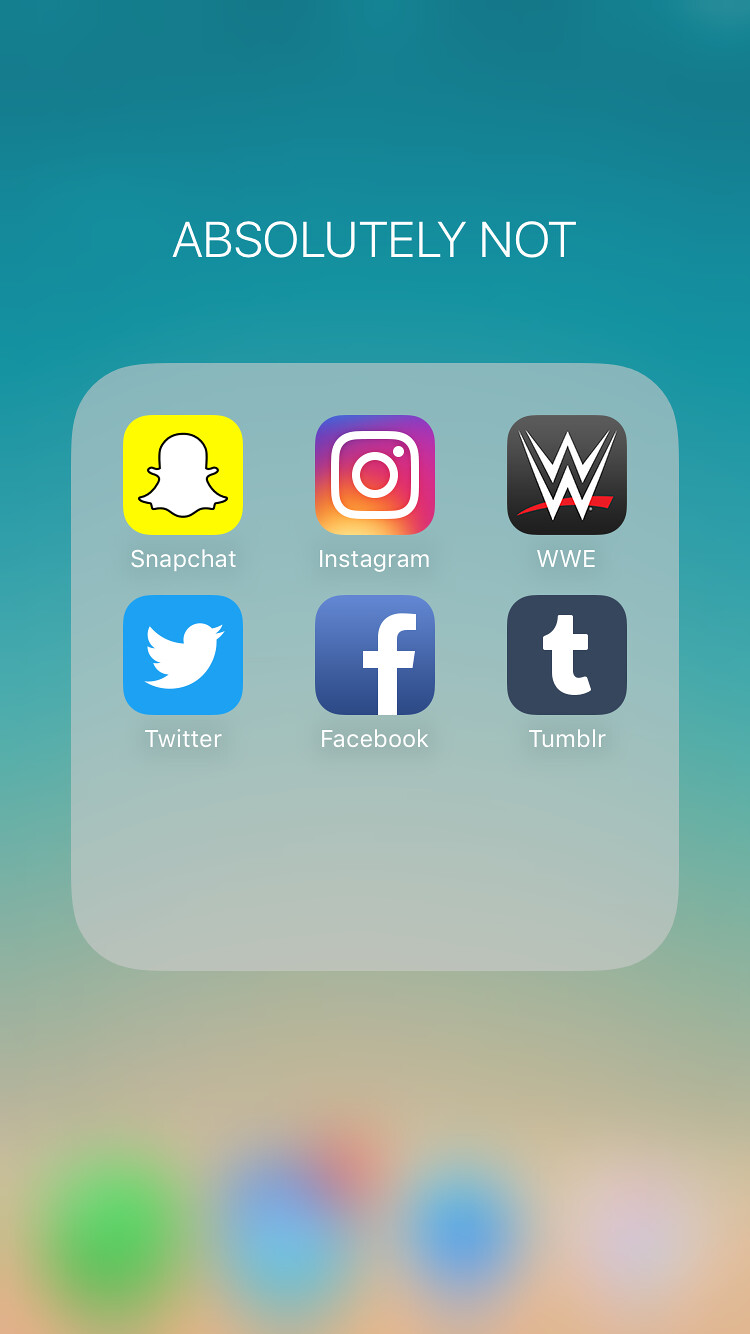A visually striking smartphone wallpaper featuring a vertically gradient background transitioning from dark teal at the top to a soft, blurred orange hue at the bottom. The gradient showcases an ombre effect, where the teal gradually lightens as it descends, creating a smooth, seamless color shift. At the top, crisp white uppercase text boldly declares "ABSOLUTELY NOT." Underneath this text, a rounded gray square icon frames six popular app logos: Snapchat, Instagram, WWE, Twitter, Facebook, and Tumblr, categorizing them under the "ABSOLUTELY NOT" directive. This composition craftily merges aesthetic gradients with a humorous, defiant message against these social media platforms.